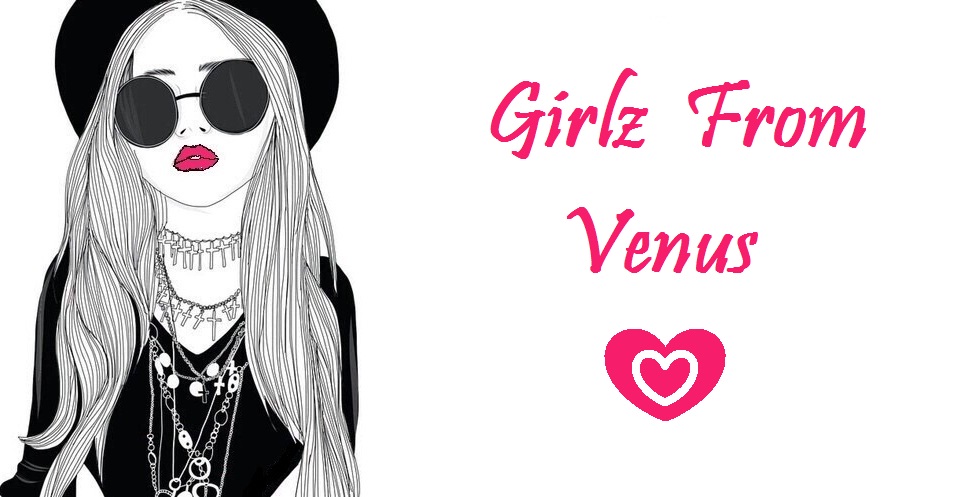The image is an illustration on a white background, portraying a close-up, black-and-white drawing of a young woman on the left side. She has long blonde hair, a black hat, and circular black sunglasses. Her lips are painted a dark red, matching the hot pink text in the image. She wears a black, long-sleeve V-neck shirt and is adorned with numerous necklaces—two of which are chokers with crosses, in addition to several beaded chains. To the right, in bright pink letters, the text "Girlz from Venus" is prominently displayed, with "Girlz" spelt with a "Z". Below the text is a large pink cartoon heart containing a smaller white heart within it.